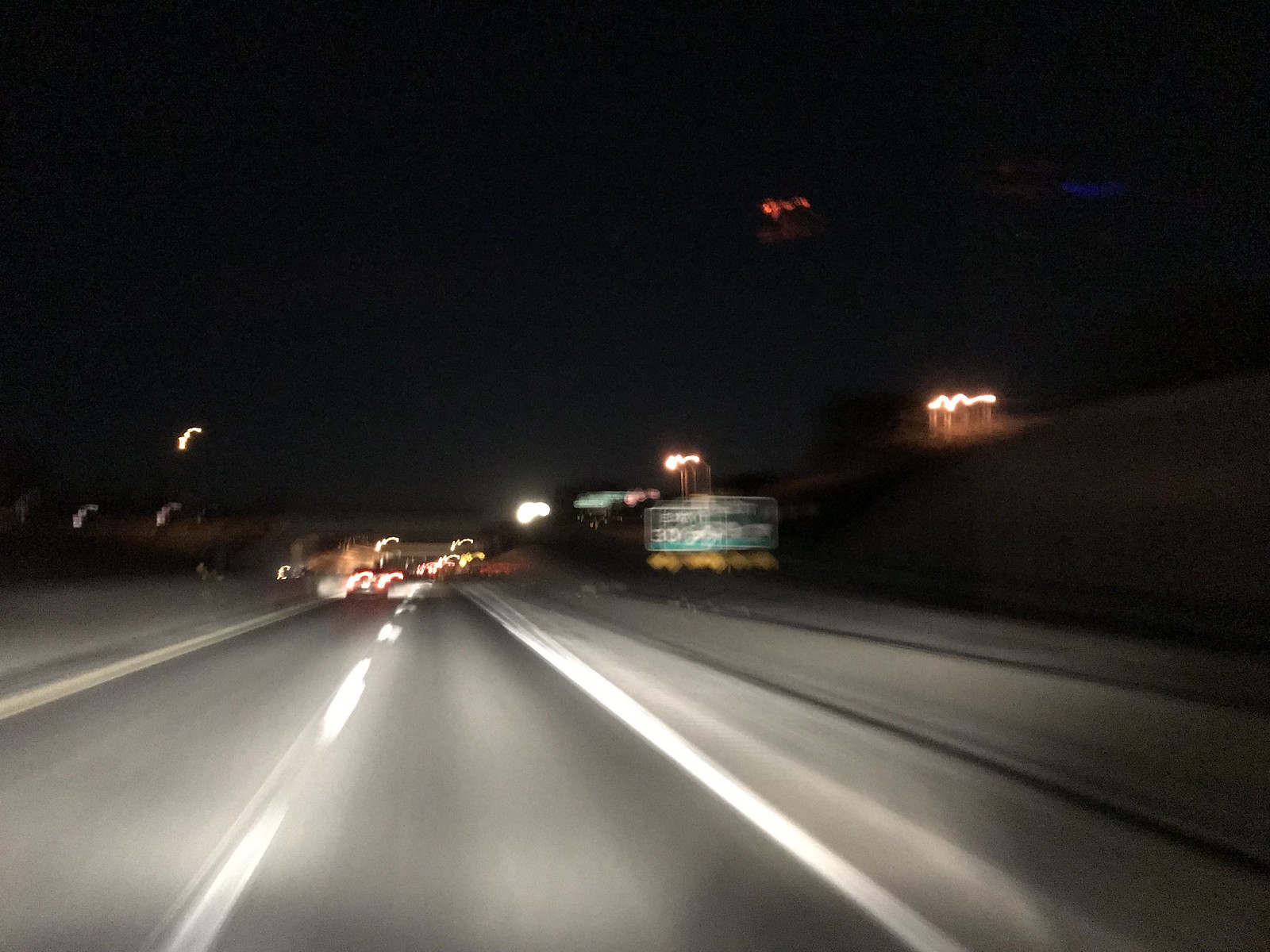The photo captures a nighttime scene on a highway. The sky above is an intensely dark blue, approaching black. On the right side of the image, there are indistinct red reflections that appear to scatter across the scene; their source is unclear. Dominating the image is a somewhat blurry highway, which becomes more indistinct as it recedes into the background. 

On the right side of the highway, there is a retaining wall of indeterminate color, behind which numerous yellow lights are visible. Also on the right side, a green exit sign with white lettering is visible, though the text is unreadable due to the image’s blurriness. 

The road itself features gray concrete barriers on both sides, bordering the asphalt roadway. The road is demarcated by two solid white lines on either side, with evenly spaced white dashed lines separating the two lanes. In the distance, an array of red taillights from several cars can be seen, though their details are obscured by the darkness and blurriness of the photo.